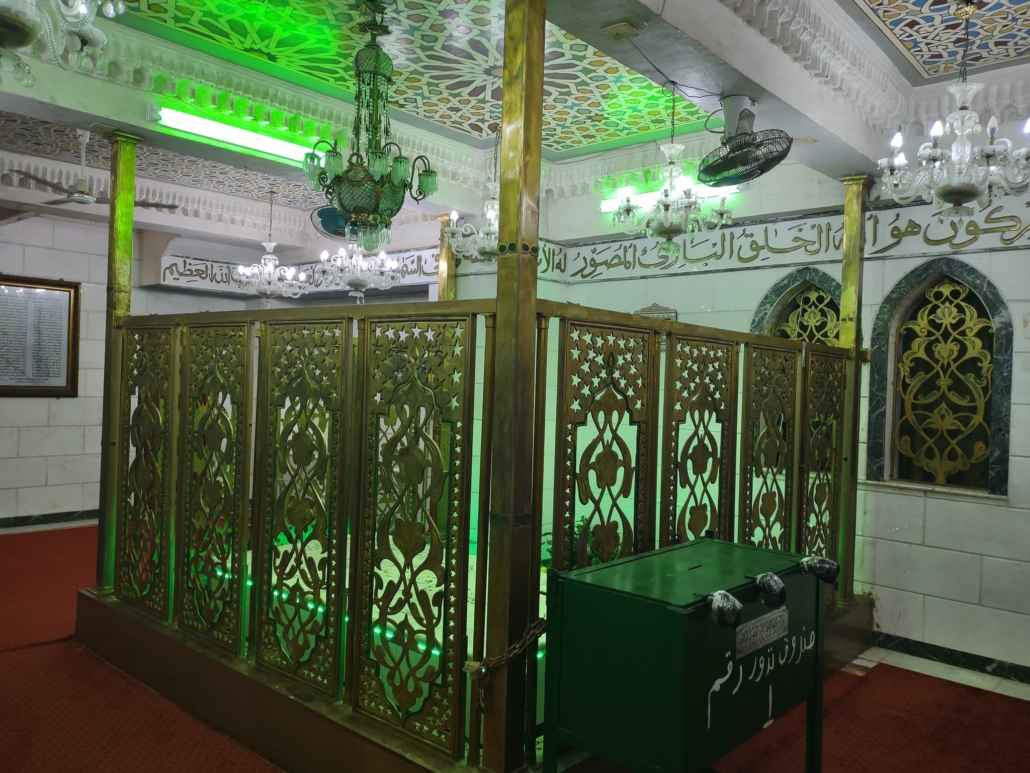The photograph captures the interior of a religious building adorned with detailed elements. The upper portion of the wall features a decorative border inscribed with religious scripture in a foreign language, elegantly framed against the backdrop of white brick-patterned tiles. The white tiles are meticulously arranged, creating a serene and structured appearance. Side windows, embellished in black and gold, add a striking contrast to the predominantly white interior. Suspended from the ceiling in the center of the room is a metallic, boxed-in compartment, suggesting a functional or ornamental role. Above, glowing neon green lights cast a vibrant illumination, adding a modern touch to the sacred space. Additionally, numerous white chandeliers hang gracefully from the ceiling, their bright and uniform design contributing to the overall luminosity and reverence of the environment.